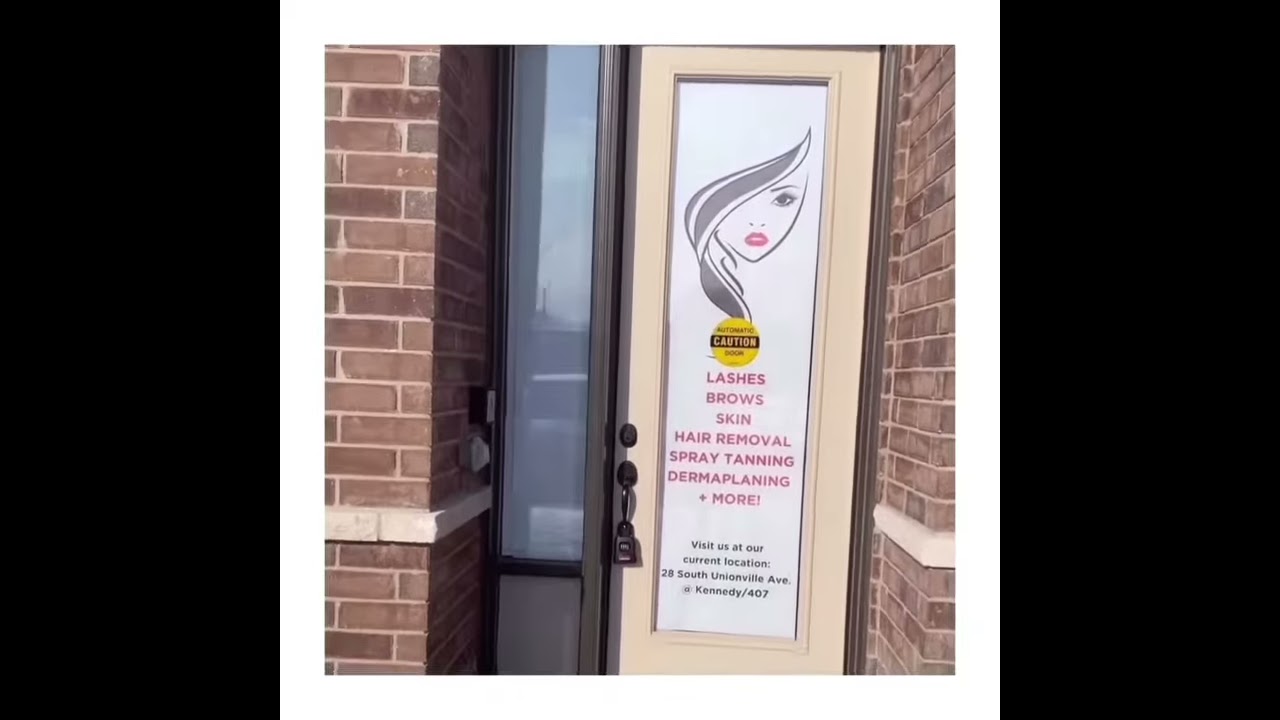The image is a photorealistic or photographic capture of a brick building, slightly off-center and angled. Dominating the composition is a narrow door with a gray-black frame and a light brown color, situated slightly to the right of center. The door features a prominent large white panel with various elements. At the top of this panel is a stylized graphic of a woman's face, with only one eye, her nose, and mouth visible, partially obscured by flowing black hair. Below this graphic, there is a yellow and black caution sign indicating "Automatic Door." Further down, in pink text, the services offered are listed: "lashes, brows, skin, hair removal, spray tanning, dermaplaning, plus more!" Below this, in smaller black text, reads: "Visit us at our current location: 28 Unionville Avenue, Kennedy/407."

The door is equipped with a black handle and lockbox. Flanking either side of the doorway are walls made of brown, multicolored bricks. To the left of the door, a larger glass panel is visible but obscured by an internal covering. The photograph is framed within a white rectangular border, with additional narrow black rectangles outside this frame, emphasizing the central focus of the doorway and its detailed signage.